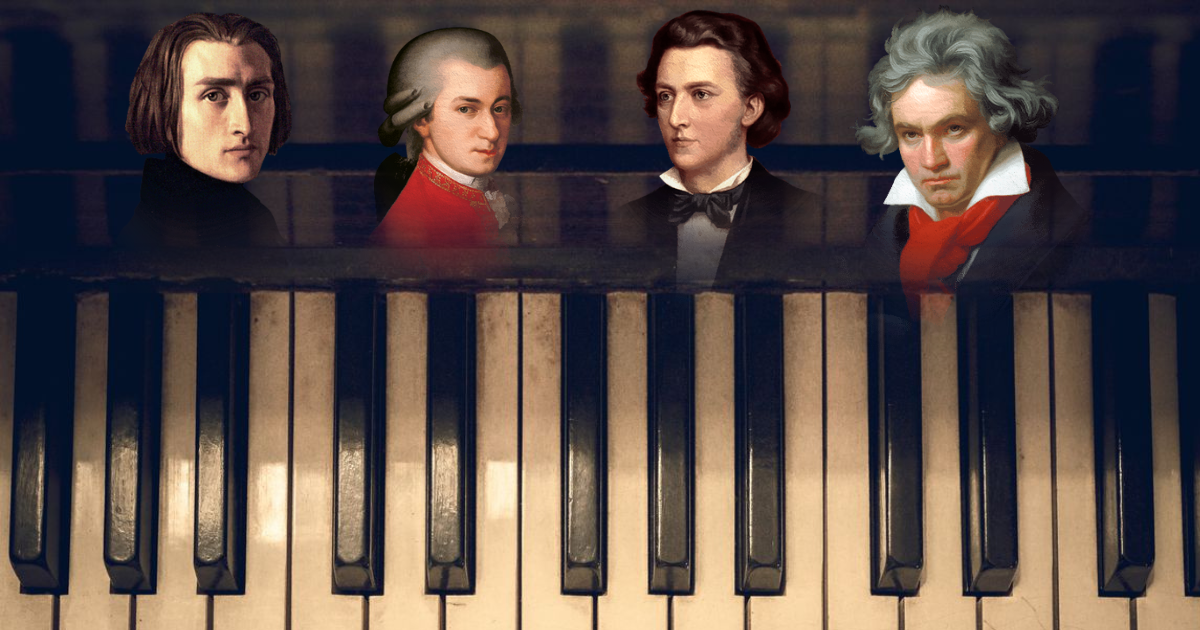The image features a close-up of an old piano keyboard, showcasing 20 white keys interspersed with 12 black keys. The keys appear dirty, indicating the piano's age and need for cleaning. Above the keyboard are portraits of four men in very old-fashioned clothing, resembling famous composers. On the left is a man with brown hair down to his chin, dressed in a dark shirt. Next to him, a man with possibly braided grayish-black hair wears a red jacket. The third man sports curly brown hair, a black jacket, a white shirt, and a bow tie and appears to be in his 30s or 40s. The fourth man, likely Beethoven, has bushy gray hair, a black jacket, a white shirt, and a red ascot. The men are not smiling; their expressions are somber as they look forward. None of the portraits are labeled, leaving the identification of these individuals open to interpretation.